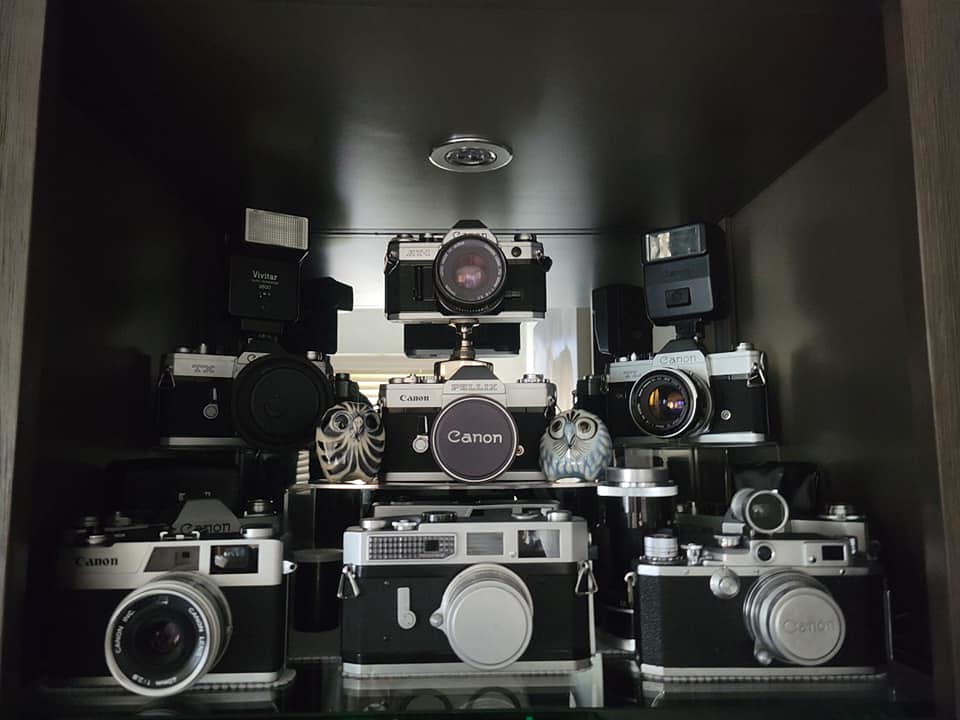This photograph captures a meticulously arranged, tiered display of Canon cameras set within a cube-shaped, black display case, likely seen through a store window or in a museum exhibit. There are seven cameras in total, varying in type and likely from different eras. The display is structured in three rows: three cameras at the front on ground level, three in the middle row on slightly raised risers, and one at the top on the highest riser. Additionally, there are two large black housing flashes, one behind the middle row cameras and another to the left. Two of the cameras at the bottom row have their lens caps on. The overall color scheme emphasizes black and silver. Nestled among the middle row cameras are two black and white ceramic owls. Though the case includes a light fixture, it is currently turned off. This scene was captured by a passing photographer during the day, adding a natural light focus to the display.